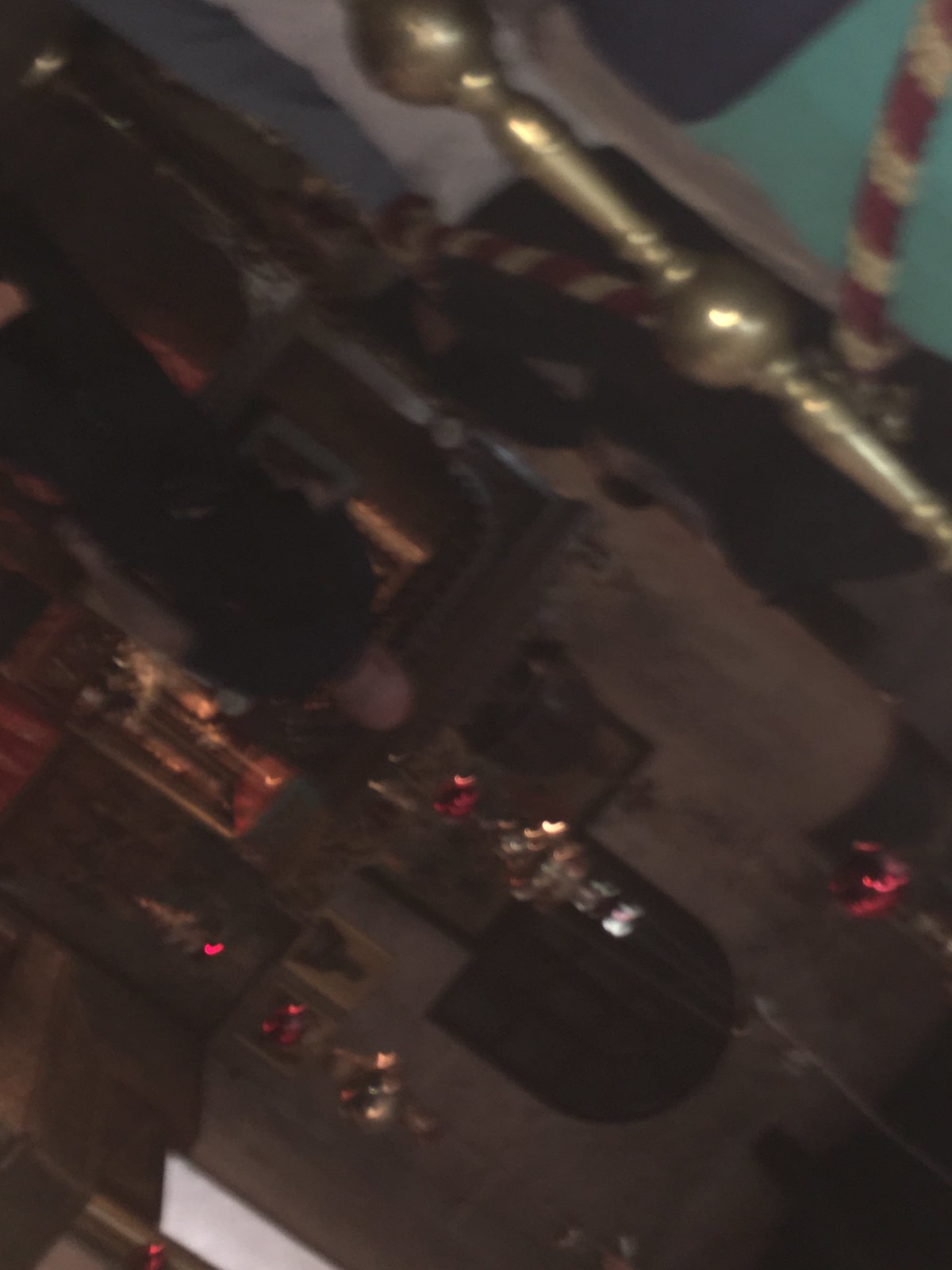This upside-down, color photo captures the dimly lit interior of a church, making it challenging to distinguish details. Central to the image is a bald, black-clad man standing at the altar. The church's walls feature hanging decorative lights in gold and red hues, and a few pictures adorn them. In the bottom left corner, there's a visible brass leg, and a red and white striped rope stretches across this section. Despite the photo's blur and darkness, hinting at the richness of the architectural details, such as gold accents and a curved wooden window. The environment seems to blend concrete and possibly wooden elements. An orange and black light adds to the overall ambiance.